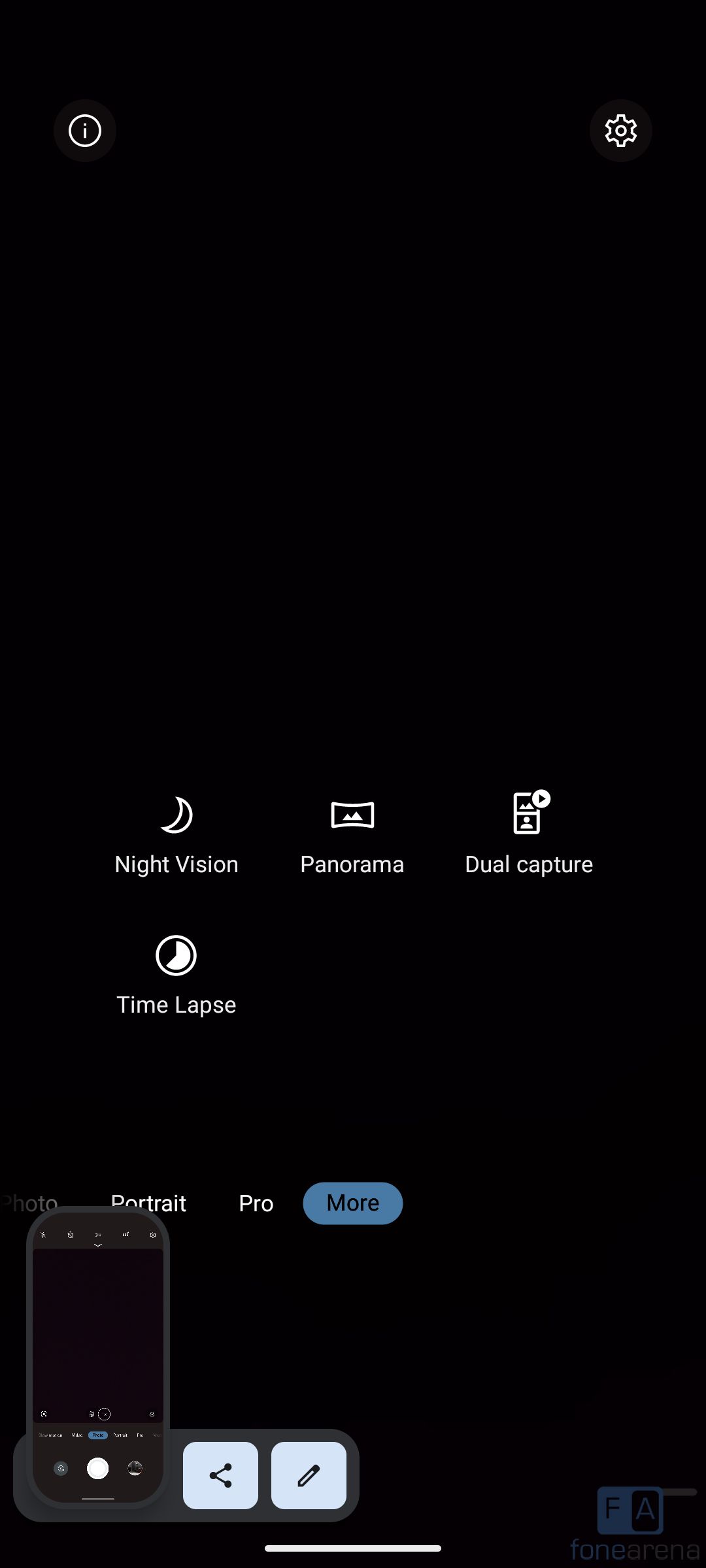The image depicts a detailed illustration of a smartphone screen positioned upright in profile orientation. The primary feature is a black rectangular screen, purposefully shaped with squared corners to resemble a phone. In the bottom left corner of this screen is a smaller, more detailed illustration of another smartphone. This secondary phone graphic has rounded edges and displays familiar icons and a white button, mimicking the look and feel of an actual phone display.

At the top right of the main screen, several icons are aligned in a row: a settings gear icon, an information 'i' icon, and labels for different camera modes, including "night vision," "panorama," and "dual capture." Below this row is another line featuring a "time lapse" icon. The third line displays the words "Portrait Pro," with a prominent blue button labeled "more" directly beneath it. The small superimposed phone illustration is proportionally tiny compared to the larger screen, reinforcing the layered visual concept of a "phone within a phone."